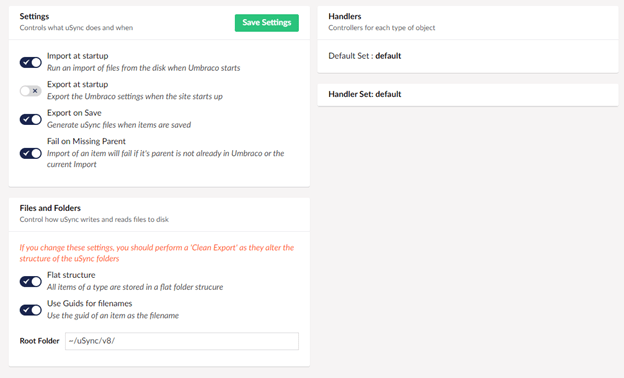This image displays a comprehensive interface for configuring the settings related to the USYNC functionalities within the Umbraco content management system. It is a user interface where users can adjust various control options for USYNC, specifying what actions it performs and when they are executed. The interface is organized under several headings with descriptive icons.

Firstly, under the "Import and Startup" section, the user can:

1. **Run an Import of Files from Disk on Startup:** This setting ensures that files are imported from disk whenever Umbraco starts.
2. **Export on Startup:** Allows the exportation of Umbraco settings automatically during the startup of the site.
3. **Export on Save:** Generates USYNC files whenever items are saved within Umbraco.
4. **Fail on Missing Parent:** Ensures that the import process fails if the item's parent is not already present in Umbraco or in the current import batch.

In this section, the interface indicates all settings are enabled except for "Export on Startup," which is marked with an 'X' to signify its disabled status.

Next, under the "Files and Folders" section, the background switches to a white area with black text. It instructs the user on how to control how USYNC writes to and reads from disk, and suggests performing a clean export when these settings are changed, as these adjustments will alter the structure of USYNC folders. The section includes:

1. **Flat Structure:** All items of a similar type are stored in a flat folder structure. This setting is enabled and marked by a checked icon.
2. **Use GUIDs for Filenames:** Uses the GUID of an item as its file name. This setting is likewise enabled, indicated by a checked icon.
3. **Root Folder:** This involves a text box where users can specify the base directory for USYNC. The text box currently shows the path “\-USYNC\-V8\-”.

At the top right of the image, the "Handlers" section provides controls for each type of object with default settings applied. This section seems to encapsulate the default setup for various handlers within the system.

Overall, the interface is well-organized, providing users with the tools to customize their USYNC integration with detailed settings presented clearly with helpful icons indicating their statuses.